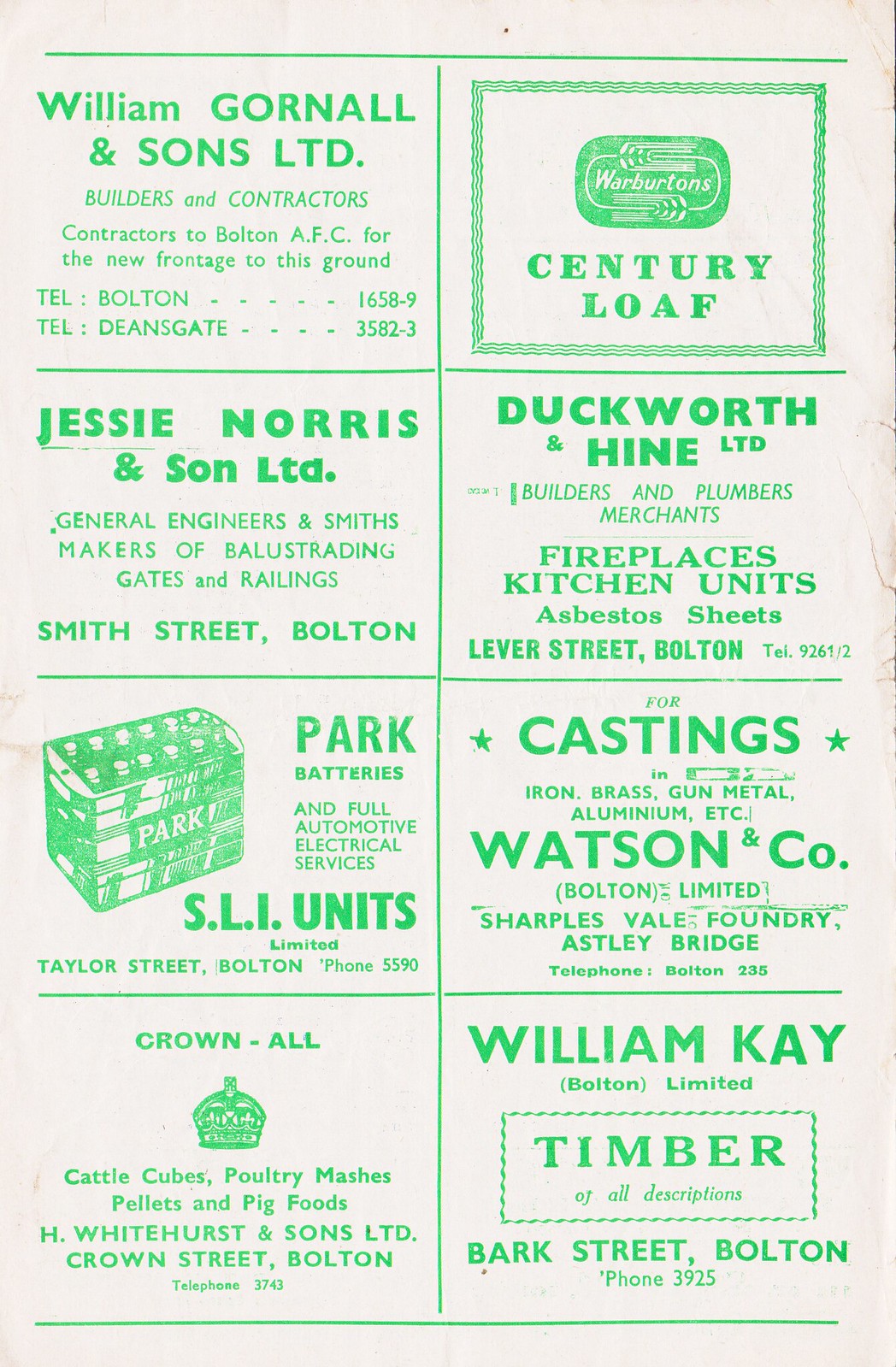This image is a scan or photograph of an old, worn magazine or newspaper page with a white background and bright green text. The page is organized into two vertical columns, each further divided into four sections, making a total of eight distinct advertisements. 

Starting from the top left, the first advertisement reads "William Gornall & Sons Ltd. Builders and Contractors," with additional information below. Directly beneath it, the next ad is for "Jesse Norris & Sons Ltd. General Engineers and Smiths, Makers of Balustrading, Gates, and Railings, Smith Street, Bolton." The third ad on the left features an artist’s illustration of a battery and reads "Park Batteries and Full Automotive Electrical Service SLI Units." At the bottom left, there is an ad with an illustration of a crown labeled "Crown All: Cattle Cubes, Poultry Mashes, Pellets, and Pig Foods."

In the right column, the top advertisement promotes "Warburton's Century Loaf." The second ad below is for "Duckworth & Hine Ltd. Builders and Plumbers, Merchants, Fireplaces, Kitchen Units, Asbestos Sheets, Liver Street, Bolton." The third down is for "Watson & Co.," which deals with "Castings in Iron, Brass, Gunmetal, Aluminum, etc." Finally, the bottom right ad reads "William K Bolton Ltd." with "Timber of All Descriptions" in a green box below it and "Bark Street, Bolton" further down.

The page’s aged and dingy appearance, along with the bright green color of the advertisements, suggests it may come from a vintage publication.